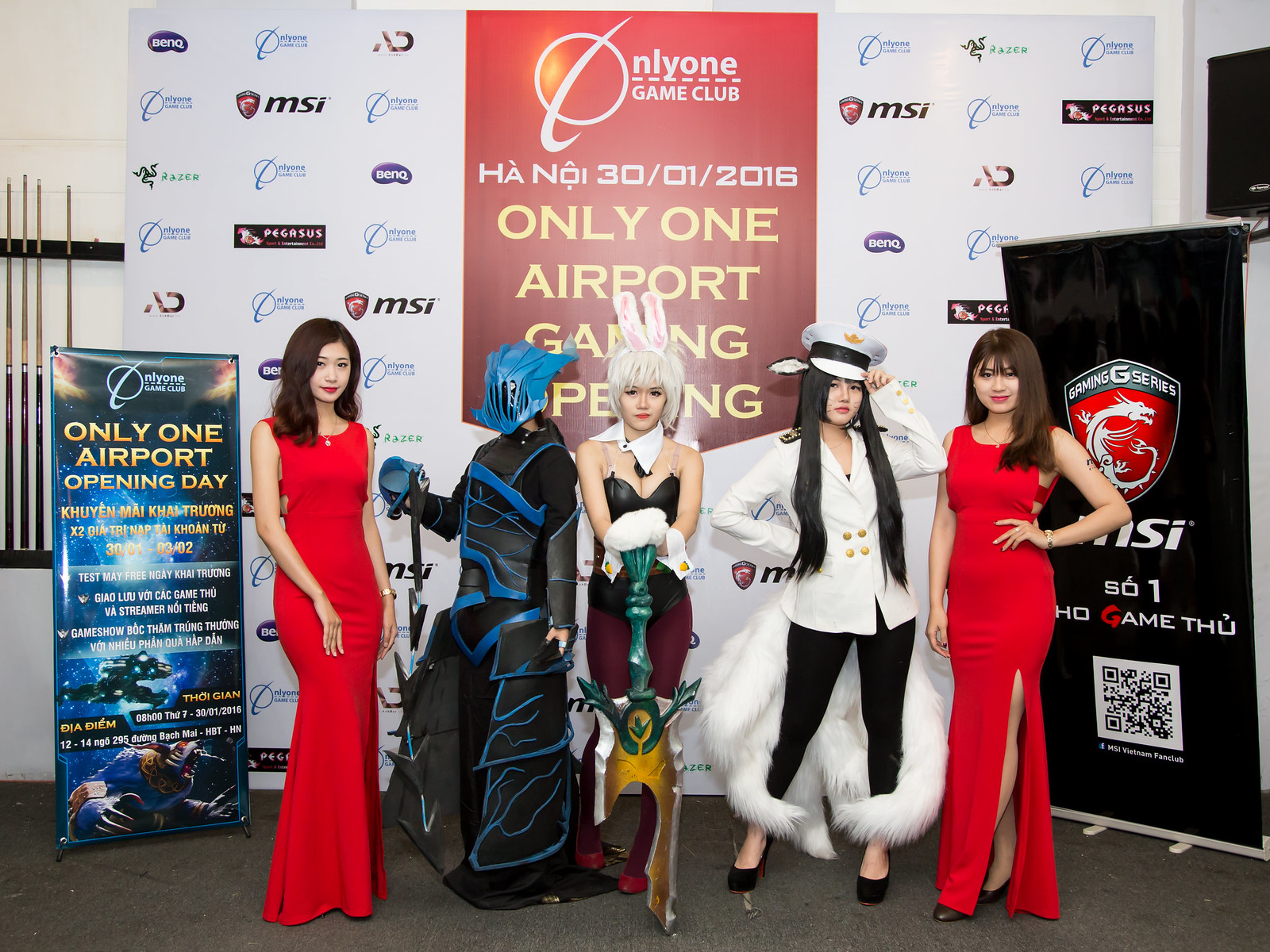In this detailed image taken at a video game convention, five women are prominently featured in front of a large press banner adorned with logos like MSI, BENQ, Razer, and Pegasus. The event's central red section reads "NLYONE Game Club. Only one airport gaming," alongside various other promotional signs, some of which appear to be in an Asian language, possibly Indonesian.

The five women are all cosplaying different characters. On the far left is an Asian woman with long dark hair, wearing an elegant red gown. Next to her stands a figure in an elaborate black and blue costume with a blue helmet and mask, covered in armor resembling lightning bolts.

In the center, an Asian woman with a blonde wig sports bunny ears, a white collar, a black bustier, and maroon pants, while holding a sword. To her right is another Asian woman with long dark hair, dressed as a ship captain in a white double-breasted blazer and black leggings, accented with a ship captain's hat and large white wings draped around her legs.

On the far right, matching the first woman, is another woman in a red gown, with long brown hair. The backdrop also features "Gaming G-Series" on a separate black sign, and other phrases like "Only one airport opening day" can be seen partially obscured behind them. The cohesive elements and themed attire confirm the atmosphere of a lively gaming event.